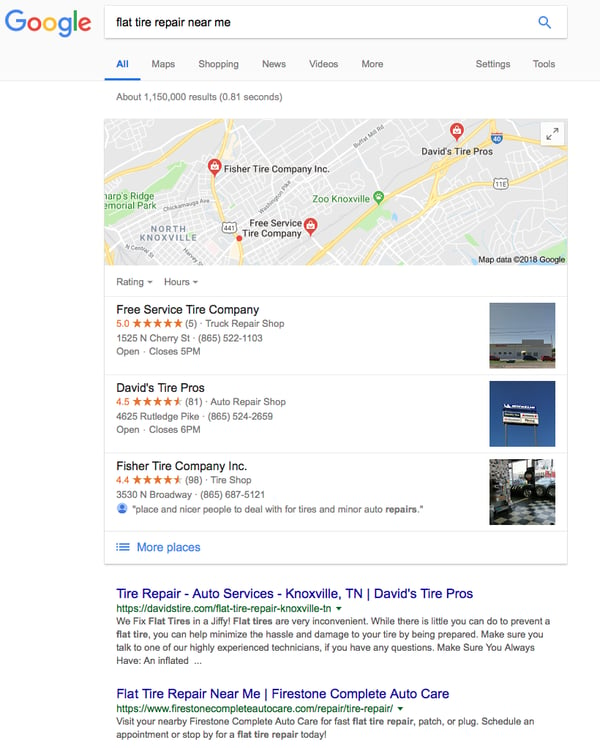In this screenshot, we observe a Google search query for "flat tire repair near me." The interface displays several interactive tabs beneath the search bar, including options such as "All," "Maps," "Shopping," "News," "Videos," and "More." On the right side, there are links to "Settings" and "Tools." 

Below the search bar, a map appears, populated with location markers indicating various tire repair services. Accompanying the map are detailed descriptions of nearby businesses:

1. **Free Service Tire Company**: Rated 5 stars, it includes the company's address and closing time.
2. **David's Tire Pros**: This business has a rating of 4.5 stars.
3. **Fisher Tire Company Inc.**: It holds a rating of 4.4 stars.

Additionally, search results include web links: 
- One of them is from davidstire.com, advertising "Tire Repair Auto Services" in Knoxville, Tennessee, specifically highlighting David's Tire Pros.
- Another listing is "Flat tire repair near me - Firestone Complete Auto Care," which features Firestone's website address.

The screenshot effectively conveys a range of options for tire repair services, complete with ratings, addresses, and additional web resources.